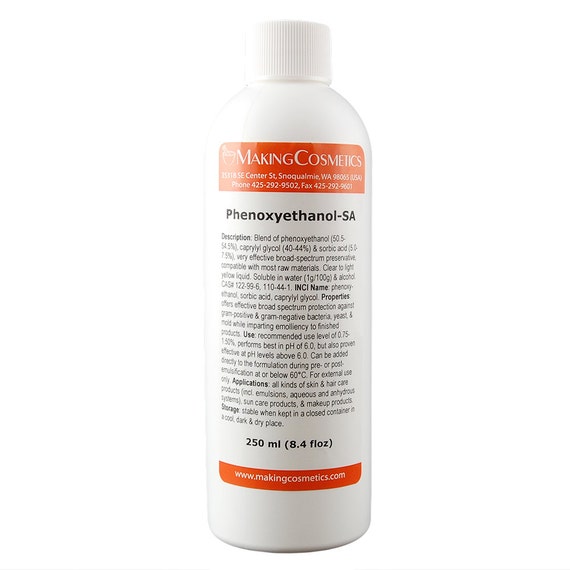This image is a detailed product photo of a white plastic cosmetic bottle with a grooved screw-on cap, standing upright against a solid white background. The bottle features a label with distinct orange bands at the top and bottom. The top orange band contains white text that reads "Making Cosmetics" along with the company's address in Snoqualmie, Washington, and a phone number, 425-292-9502. Below that, in bold black sans-serif text, the name "P-H-E-N-O-X-Y-E-T-H-A-N-O-L-SA" is prominently displayed. Following this, there is a substantial block of descriptive text in black, detailing the ingredient's properties, applications, and usage instructions. Near the bottom of the bottle, it specifies the volume as "250 milliliters (8.4 fluid ounces)" in larger black text. The bottom orange band features the website "www.makingcosmetics.com" in white text. This comprehensive label almost covers the entire body of the bottle, providing a thorough overview of the product.